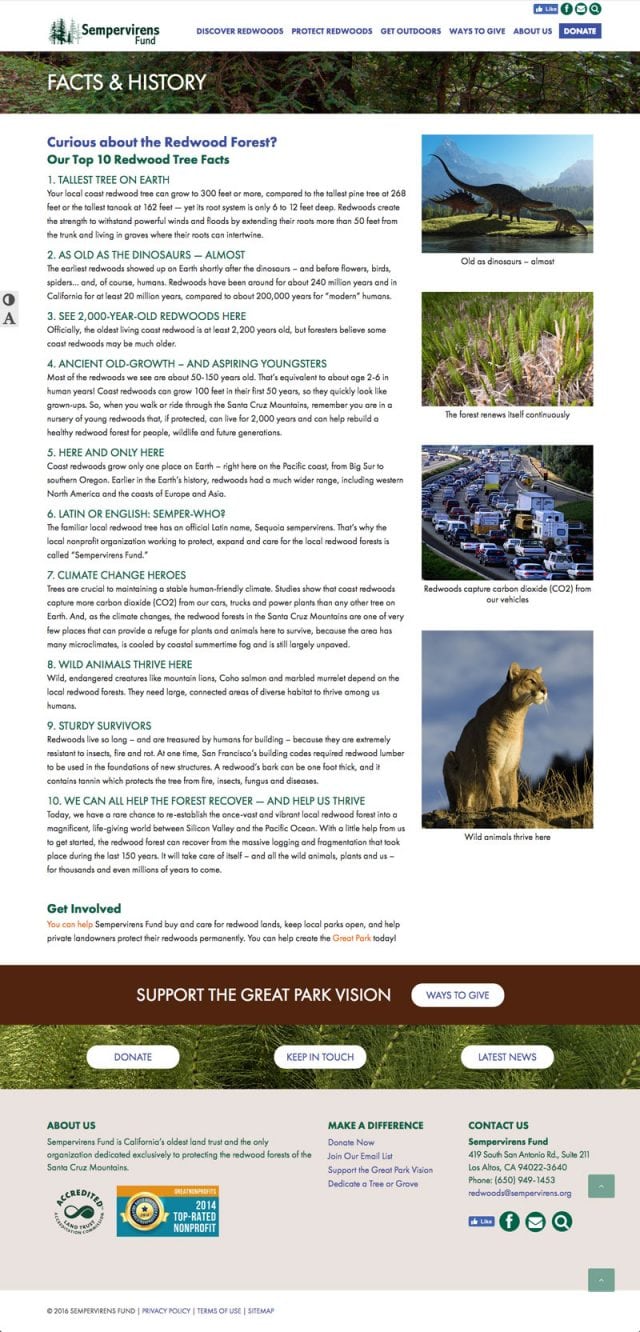**Screenshot of the Semper Varens Fund App Interface**

The screenshot showcases the main interface of a mobile application for the Semper Varens Fund. At the very top of the screen, there is a banner image followed by the name "Semper Varens Fund." Below the banner, a navigation bar presents various options in multiple small-font languages. There are five clickable choices, and a sixth one highlighted in blue.

Underneath, a picturesque image, likely of a forest, adorns the screen. It features a title overlay "Facts and History." Directly below this image, an article is listed in a bulleted format titled, "Curious about the Redwood Forest? Our Top 10 Redwood Tree Facts."

The list includes detailed points:
1. Tallest tree on earth
2. As old as the dinosaurs, almost
3. See a 2,000-year-old Redwood here
4. Ancient old growth and aspiring youngsters
5. Here and only here
6. Latin or English, Semper who
7. Climate change heroes
8. Wild animals thrive here
9. Sturdy survivors
10. We can all help the forest recover

Alongside each fact, there are corresponding images to engage the reader visually.

At the bottom of the screen, the user can select from three options to engage further with the fund: 
- Donate
- Keep in Touch
- Latest News

These options allow users to support the fund, stay updated, and contribute to their cause.